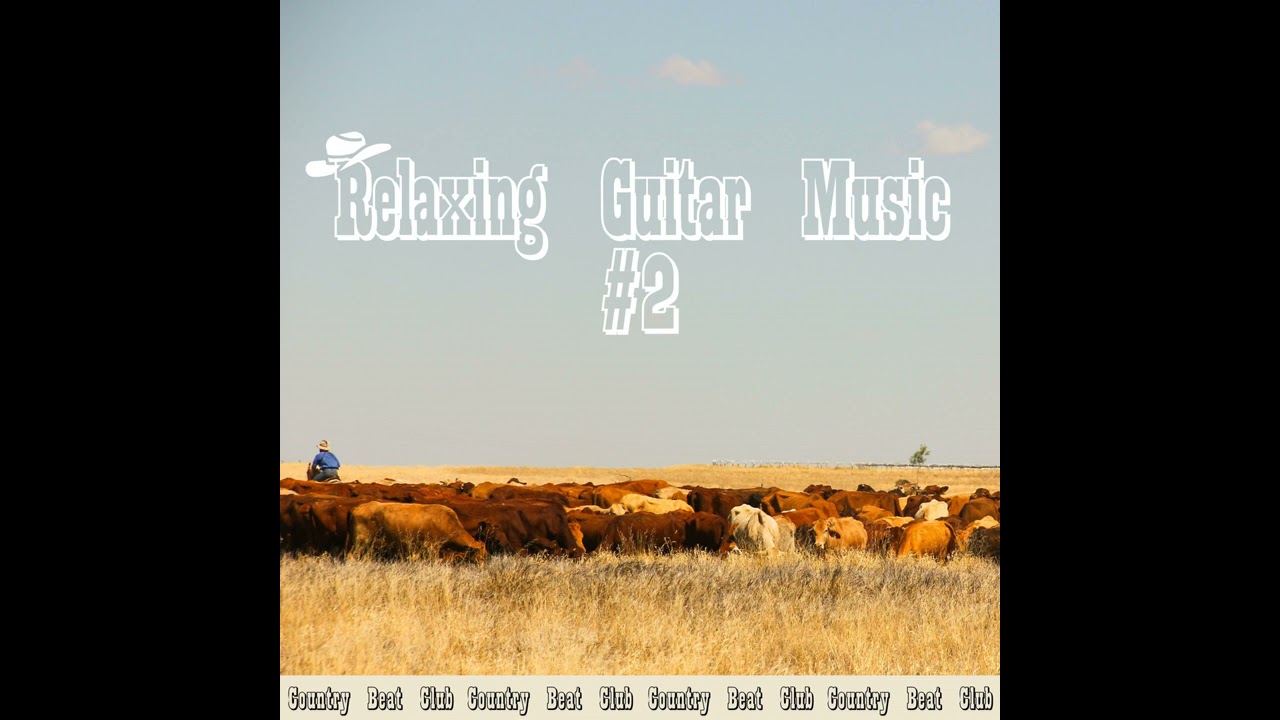The image is a detailed cover for a music album titled "Relaxing Guitar Music No. 2." Framed by black borders on the left and right, the central picture features a herd of cattle grazing on dry, yellowish grass, with the animals predominantly brown and some white. In the background, a cowboy wearing a blue shirt and cowboy hat is seen herding the cattle, with a tree off to the right under a mostly clear light blue sky dotted with a few clouds. At the top of the image, the album title "Relaxing Guitar Music No. 2" is prominently displayed in white text, with a cowboy hat cleverly placed over the letter 'R' in "Relaxing." At the bottom of the cover, the phrase "Country Beat Club" is repetitively printed across the ground where the cattle graze. The colors in the image are primarily black, white, various shades of brown, blue, tan, and off-white, all combining to evoke a serene, pastoral scene.